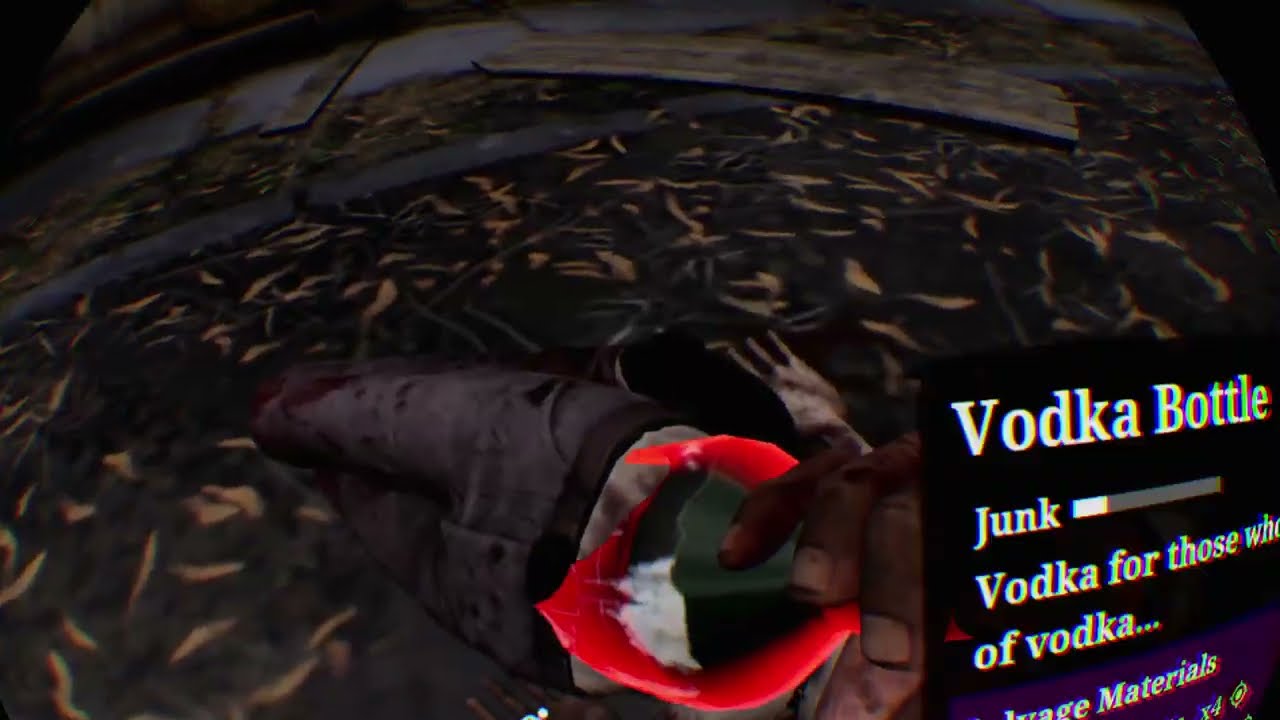The image is a digitally altered screenshot depicting a chaotic and surreal scene. On the right-hand side of the image, there is a black rectangular label with white text that reads "Vodka Bottle Junk" and "Vodka for Those Who." The text appears incomplete due to being cut off. Below the text, in a purple box, there are the words "salvage materials." The background surrounding this label is a mixture of black and purple hues. In the lower right corner, there is an eerie image of disjointed, bloody fingers seemingly gripping a fork, adding a macabre element to the scene.

The central figure in the image appears to be seated, possibly on the ground or a bench, and is drinking from a glass bottle. The person is dressed in brown pants and a white shirt. The backdrop features leafy, brown designs and a metallic silvery material at the top, suggesting a mixture of organic and mechanical elements. This gives an impression of the scene being set in a park or an industrial area. The overall color palette is distorted, adding a surreal and unsettling tone to the image.